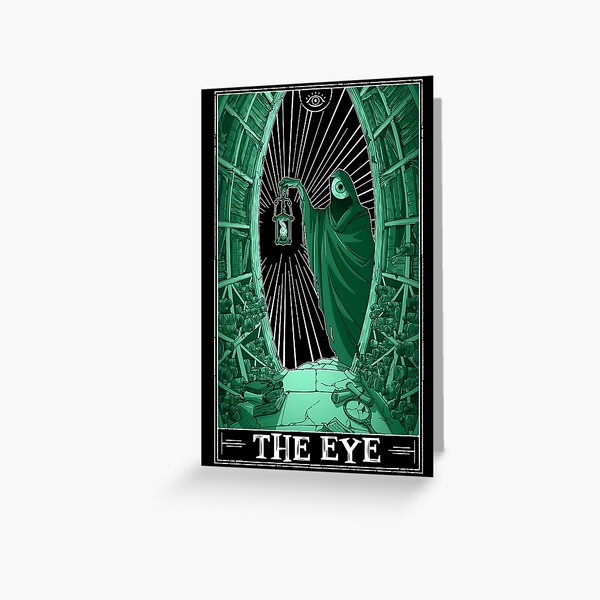This detailed description merges elements from all three captions into one cohesive narrative:

The image is a photograph of what appears to be a book cover or a card with striking artwork. The central illustration features a mysterious, green-cloaked figure standing in front of a wooden-framed doorway or portal. The figure's face is replaced by a large, staring eyeball, casting an eerie gaze directly at the viewer. The figure holds a lantern with a haunting green flame that illuminates the surrounding area. The background behind the figure is predominantly black, accentuating the eerie atmosphere.

At the top of the image, there's an additional symbol of an eye, further emphasizing the theme. At the bottom, in a bold white panel, the text reads "THE EYE" in all capital letters. The overall composition is bordered in black, adding a sense of depth and framing the central elements. The entire setup rests on a plain white background, creating a stark contrast with the dark imagery and making the green and black elements stand out vividly. Additionally, small details like a tennis racket on a cracked sidewalk add an unusual and surreal context to the scene.